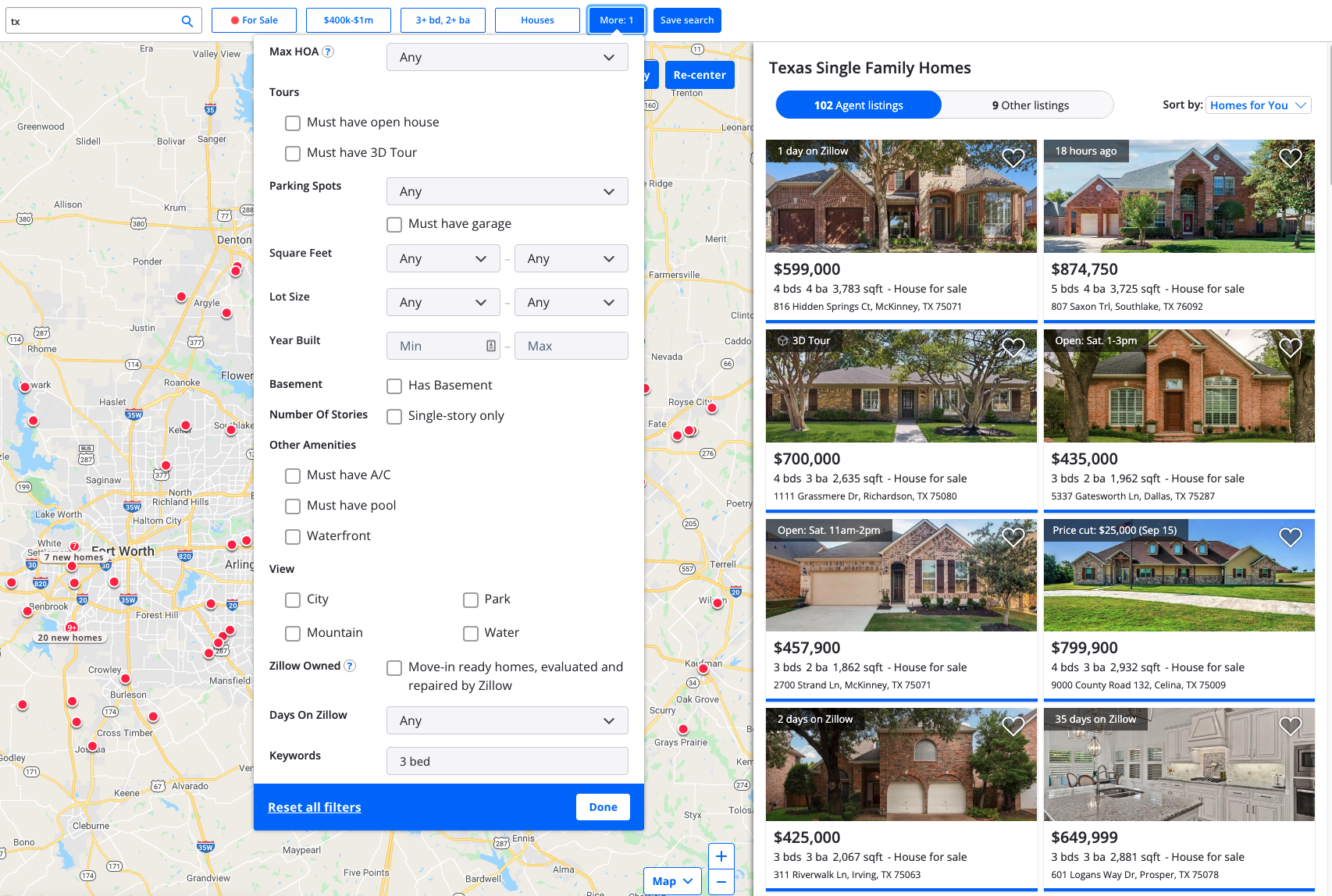The image captures a detailed screen from the Zillow website, prominently featuring a search interface and property listings. At the top left, there's a search bar with 'TX' entered, suggesting a focus on properties in Texas. Adjacent to the search bar are various filter options including 'For Sale' and 'Price', which allow users to customize their search criteria. Further to the right, buttons for adjusting 'Bedrooms' and 'Bathrooms', as well as refining 'Houses' preferences, are visible. 

The 'More' button, highlighted in blue, indicates it is currently selected and expands a dropdown menu over the map on the left side of the screen. This dropdown provides additional filter options such as 'Max HOA', 'Tours', 'Parking Spots', 'Square Feet', 'Lot Size', 'Year Built', 'Basement', 'Number of Stories', 'Other Amenities', 'View', 'Zillow Owned', 'Days on Zillow', and 'Keywords'. Users can reset all filters with a button at the bottom left, or confirm their selections with a 'Done' button on the right side.

On the right side of the image, a large white panel displays the title 'Texas Single Family Homes'. It also shows the number of agent listings, a button for 'Other Listings', and a sorting option labeled 'Sort by' with 'Homes for You' selected. Below this header section, several thumbnails of houses are presented. Each thumbnail includes a banner indicating how long the property has been listed on Zillow, with additional details and pricing located at the bottom of each image.